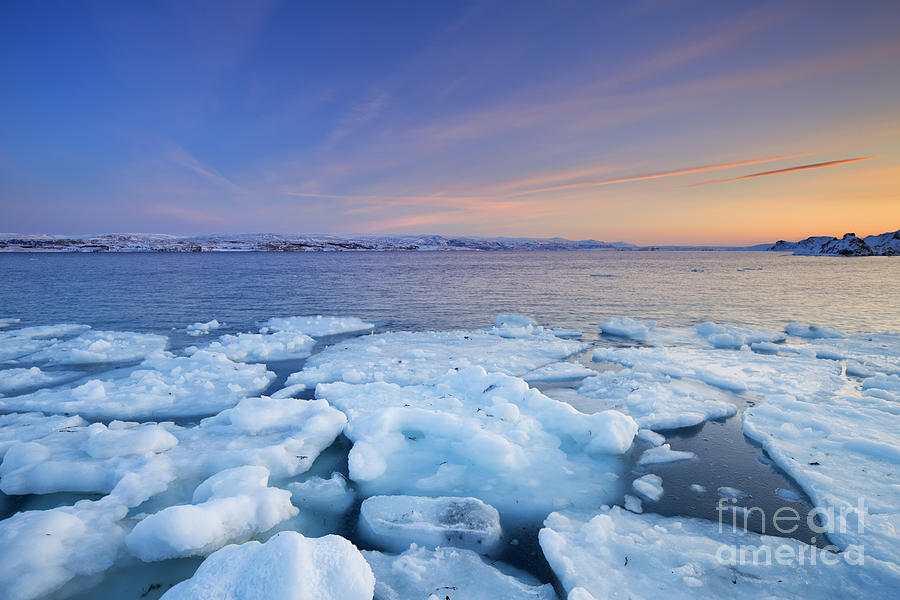The captivating image depicts what is likely a coastal scene in a region such as Alaska, Greenland, or the Arctic, characterized by prominent glacier activity and snow-covered terrain. In the foreground, sizable chunks of ice float on turquoise-tinged water, while some broken pieces hint at the disruptive effects of global warming. The extensive body of water stretches toward the horizon, where snow-capped landforms meet the sky. The land appears relatively flat with some gentle hills peeking through the snow, exposing patches of earth.

The sky overhead is a mesmerizing blend of blue with streaks of orange, red, and creamsicle hues, suggesting a brilliant sunset. Thin, high clouds add to the clarity and beauty of the scene. To the left, a city or settlement can be vaguely discerned. Adding an artistic touch, a discrete watermark in the bottom right corner reads "Fine Art America." This image's striking contrast between the vibrant, warm sky and the cold, icy landscape encapsulates the stark beauty and environmental poignancy of the moment.